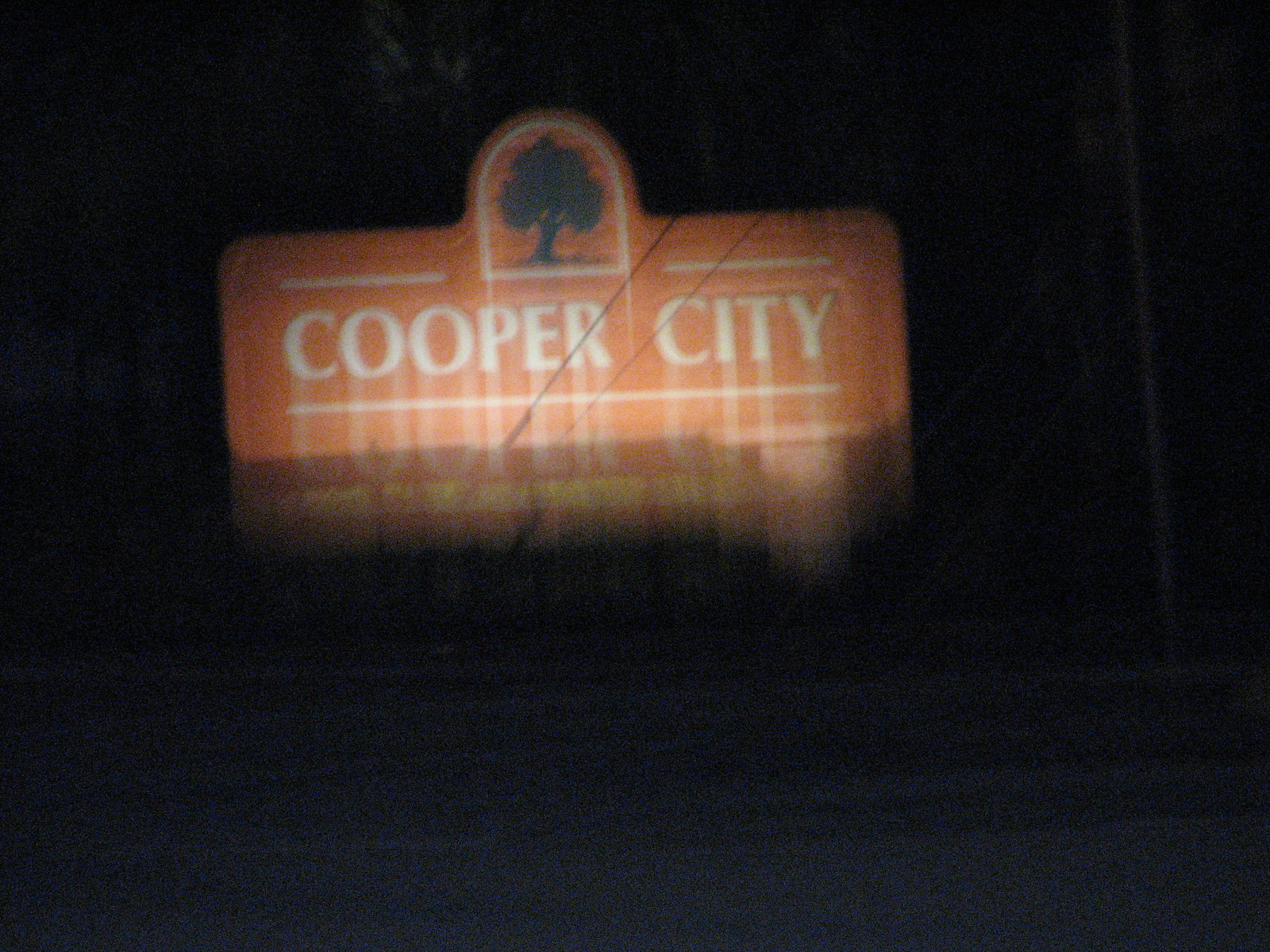Captured at dusk or night, this image showcases a distant, orange sign with the words "Cooper City" emblazoned in white letters. The poor quality of the picture gives the letters a streaking downward effect, adding a sense of movement or distortion. Behind the sign, silhouettes of trees can be seen, with faint light filtering through, highlighting the time of day. The sign also features a design of a tree in full bloom, further emphasizing its connection to nature. Below the "Cooper City" text, additional writing in yellow is present but is blurred and illegible due to the image quality. The photograph appears to be taken from a standing position, possibly on a road or a beach. To the right, a tall pole, resembling a telephone pole, is visible. The overall scene conveys a somewhat mysterious or tranquil atmosphere, captured in dim lighting.